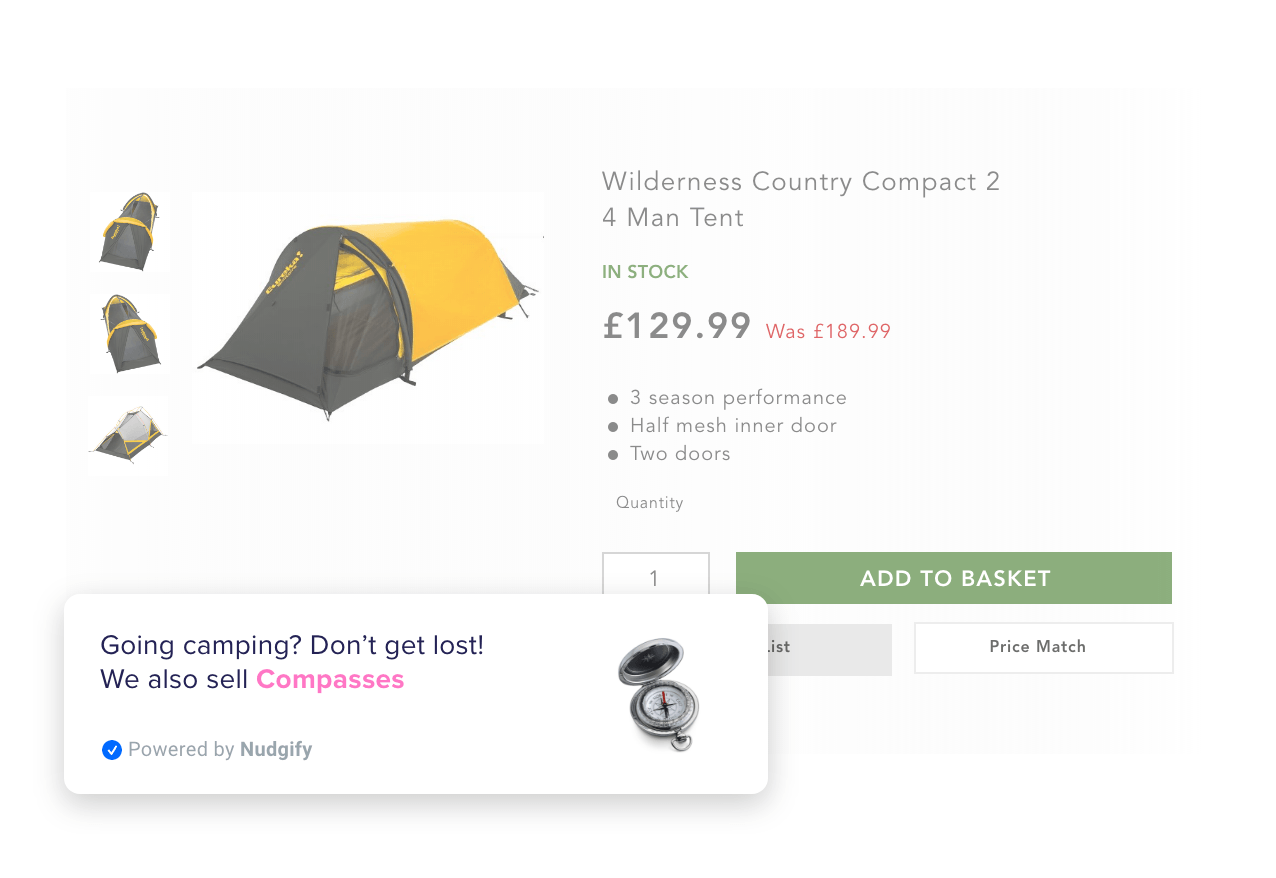The image depicts a snapshot of a retail website showcasing a camping product for sale. The featured item is a "Wilderness Country Compact 2-Man Tent," which is visually presented as a yellow and gray tent on the left side of the screen. Below the name of the tent, the site indicates that the item is "in stock" and priced at £129.99. The tent boasts "3 season performance," a "half mesh inner door," and "2 doors," making it suitable for varied weather conditions. An "Add to Basket" option is prominently displayed. 

Additionally, a pop-up advertisement appears, promoting related camping items with the message: "Going camping? Don't get lost! We also sell compasses." Accompanying the text is an image of a metallic silver or steel compass, enticing the shopper to further complement their camping gear purchase.